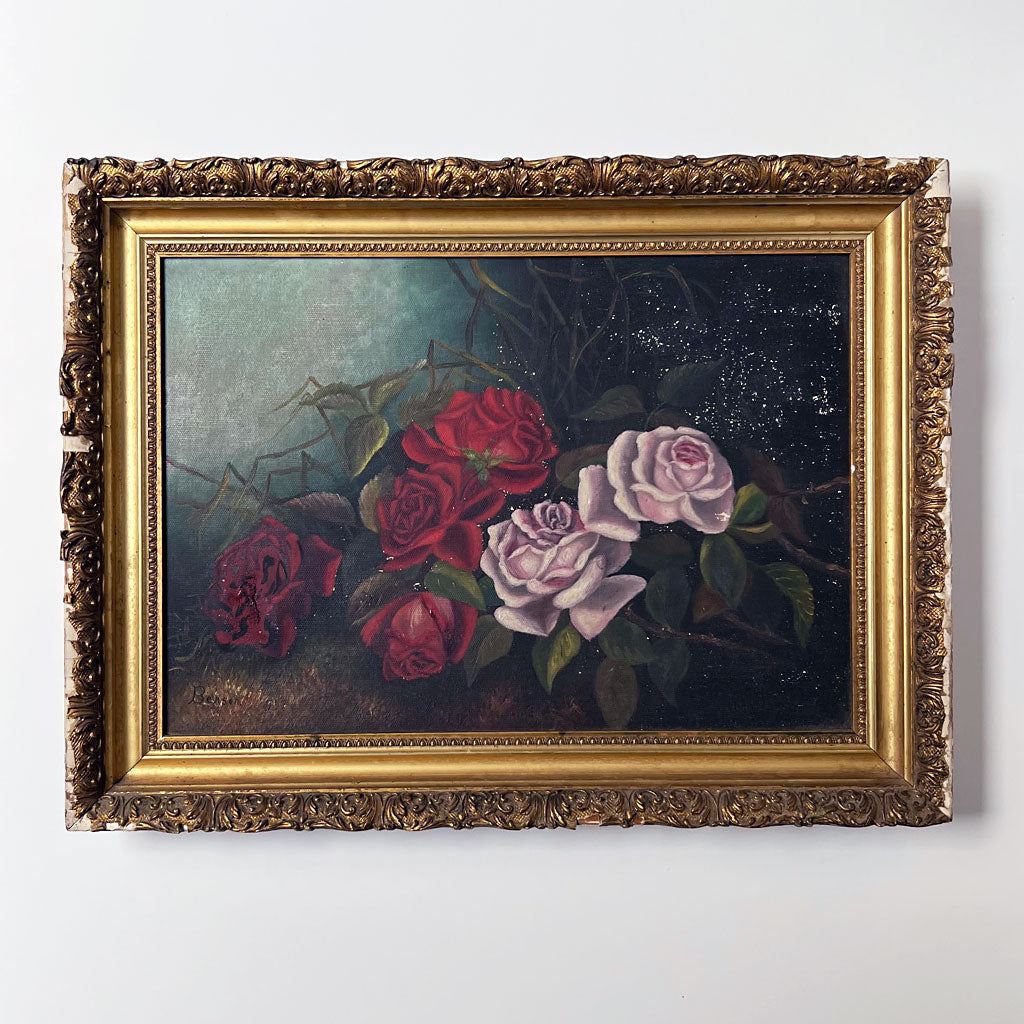A detailed oil painting hangs on a pristine white wall, encased in an ornate, gold-colored frame adorned with intricate swirls and floral designs. Some areas of the frame reveal a beige background where the gold has chipped away. Inside the gilded border, the painting showcases an array of vividly detailed roses. The composition features four deep-red roses and two pink roses, with one near-black, velvet-like rose adding depth on the far left. The green leaves and thorny stems intertwine throughout. Notably, in the upper left corner, there's an ethereal, orb-like aura blending blue, gray, and white hues, suggesting a moonlit glow. On the far right, subtle silvery glitter resembles a starry night sky. Near the bottom left of the painting, the artist's signature is visible, albeit partially obscured, appearing to contain the letters "B-E-A-S-E, peace." The overall ambiance of the artwork is dark and rich, with intricate details drawing the viewer into its enchanting floral and celestial elements.